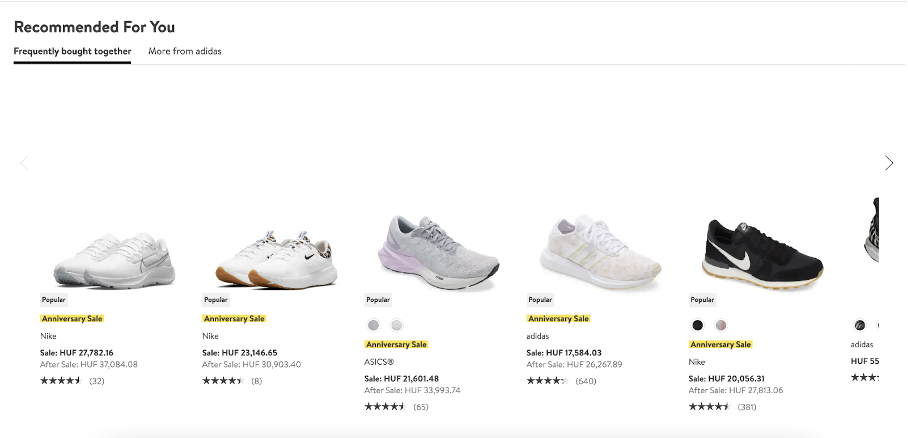In the top left corner, the image features black text reading "Recommended for You." Directly below, "Frequently Bought Together" is highlighted with underlined black text. Shifting to the right, lighter text reads "More from Adidas." Below this header section, several images of sneakers are displayed.

On the left, there is a white pair of Nike tennis shoes showcasing the iconic Nike swoosh on the side. Next to these shoes, a gray box contains the text "Popular," and next to it, a yellow tab is outlined with "Anniversary Sale." These Nike shoes have received a perfect rating of five out of five stars.

To the right, another pair of white Nike sneakers is also part of the "Anniversary Sale." The subsequent sneakers are primarily gray with accents of light purple and white; the brand is ASICS. This pair is also marked with a gray "Popular" box and included in the "Anniversary Sale."

Next, an Adidas shoe is displayed, characterized by a light gold color with white stripes on each side and labeled "Sale." Finally, a black Nike tennis shoe with a white swoosh is shown. This shoe is available in black and white color options and is part of the "Anniversary Sale," highlighted by a yellow rectangle. The text indicates "Nike Sale Huff," with a substantial quantity of 20,056 reviews and a rating of four and a half out of five stars.